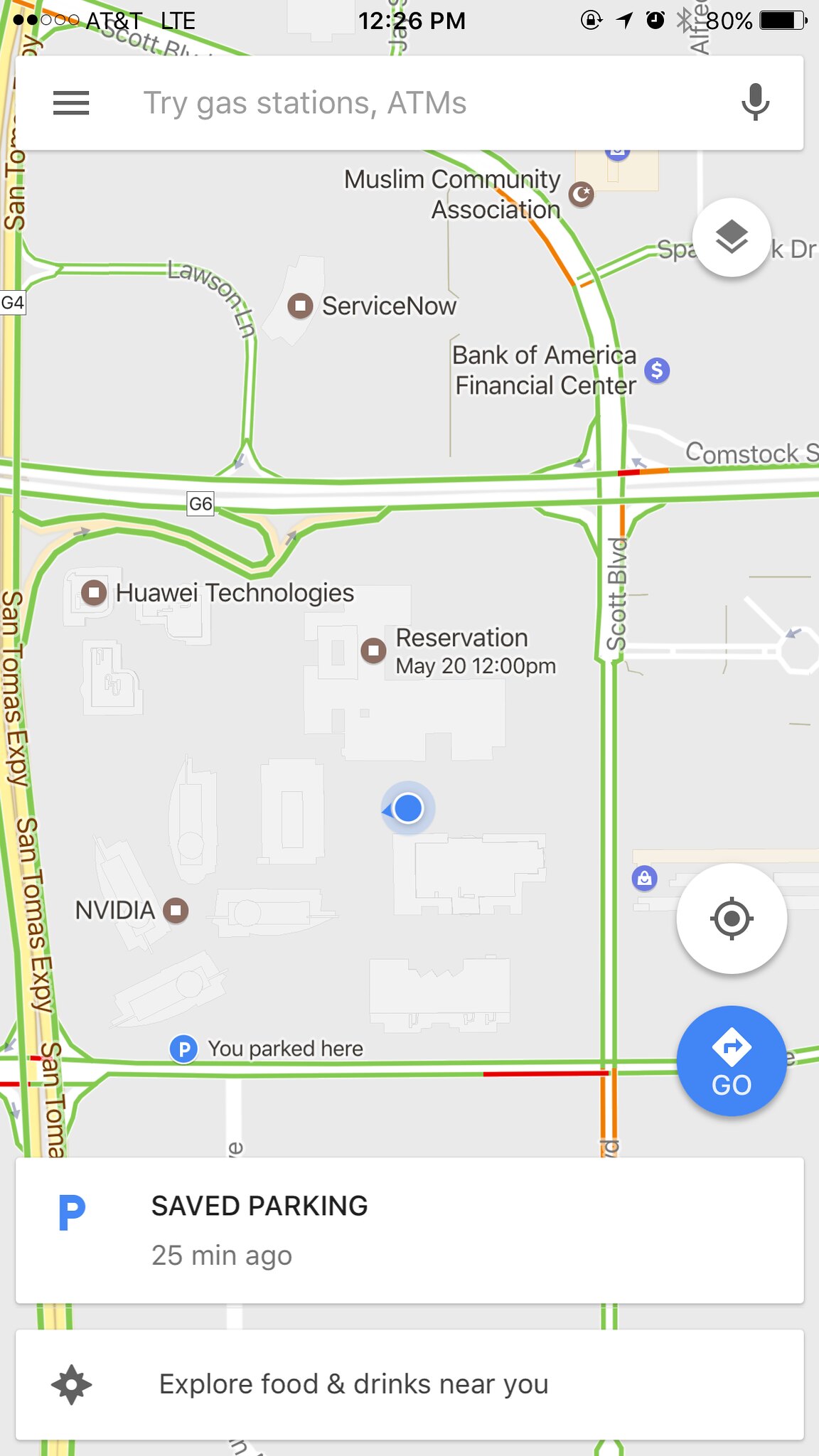This screenshot, captured from a smartphone, displays a navigational interface showing a map where a saved parking location is indicated. The map notes that the parking spot was saved 25 minutes ago, marked with a prominent blue "P" symbol both in the map legend and on the map itself. Accompanying the blue "P" icon, text reads "You parked here," pinpointing the exact location of the parked car. Surrounding this highlighted area, street names such as Scott Boulevard, Comstock Street, and the San Tomas Expressway are clearly visible, aiding in orientation. This detailed visual guide ensures easy retrieval of the vehicle by providing precise location details and identifiable landmarks.